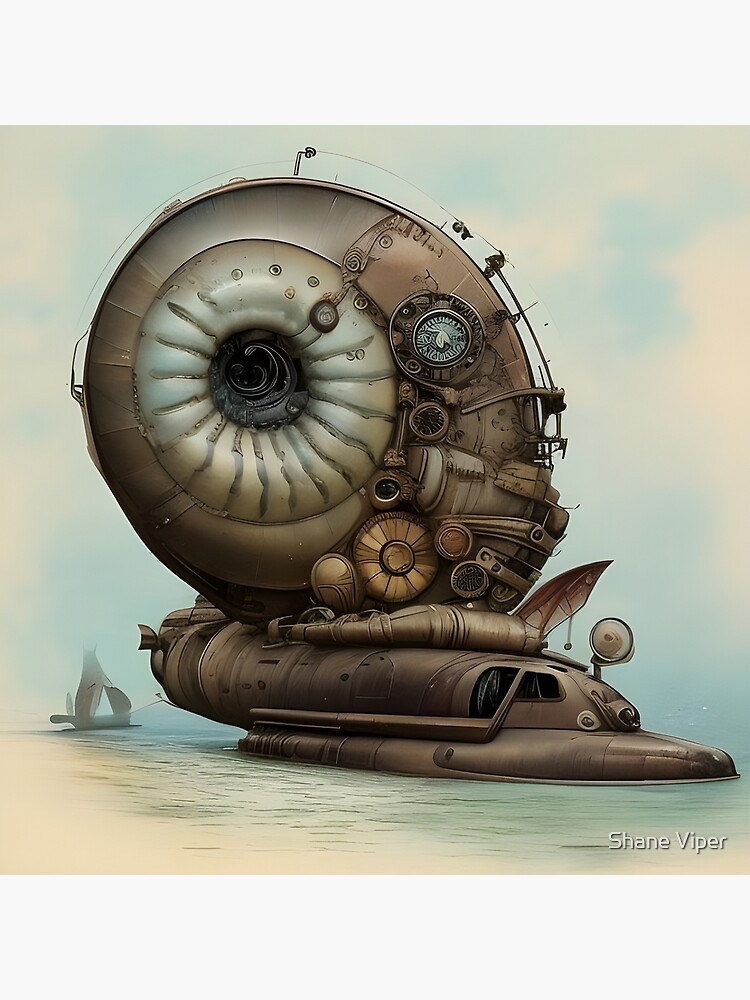This image is a highly detailed, computer-generated artwork with a cartoony and futuristic vibe. It showcases a steampunk-style, aquatic vessel parked at the seashore, featuring a blend of browns, tans, and copper hues. The vessel’s design is intricate and unique, with its primary structure resembling a submarine but incorporating elements of an airplane, giving it an unusual, hybrid appearance. Dominating the vessel is a large mechanical shell, spiral and snail-like, composed of various metallic objects with circular shapes and ridged lines, enhancing its steampunk aesthetic. Attached to this main vessel, a smaller boat with a sail can be seen, trailing behind. The sky above is partly cloudy with patches of blue visible. The bottom of the image features the name "Shane Viper" in white lettering, indicating possibly the artist or the character associated with this imaginative scene.